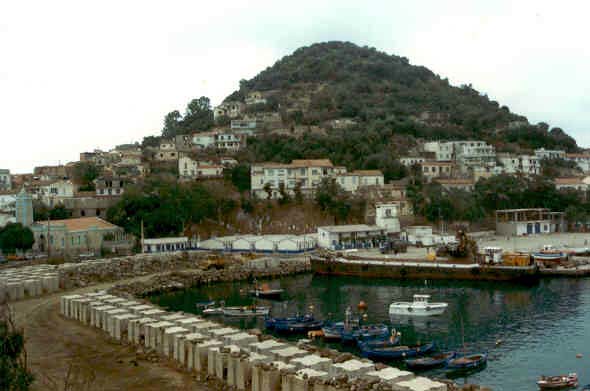This is a detailed color photograph in landscape orientation, showcasing a coastal marina set against a hillside backdrop adorned with numerous houses and apartment buildings, characterized by their large white stucco exteriors and red tile roofs. The scene features a small dock prominently positioned near the bottom, beside a dirt path that curves from the lower left toward the center of the image, bordered by white concrete pillars. The dock area is surrounded by a deep blue lagoon, populated with about seven to eight boats, most of which are docked. A single white boat is seen heading out to sea, while another boat appears to be approaching the dock. Additionally, a long, open canoe-like boat without a hood can be spotted on the other side of the dock. The overall composition captures the realistic essence of the marina and hillside housing area, emphasizing the picturesque and serene coastal landscape.